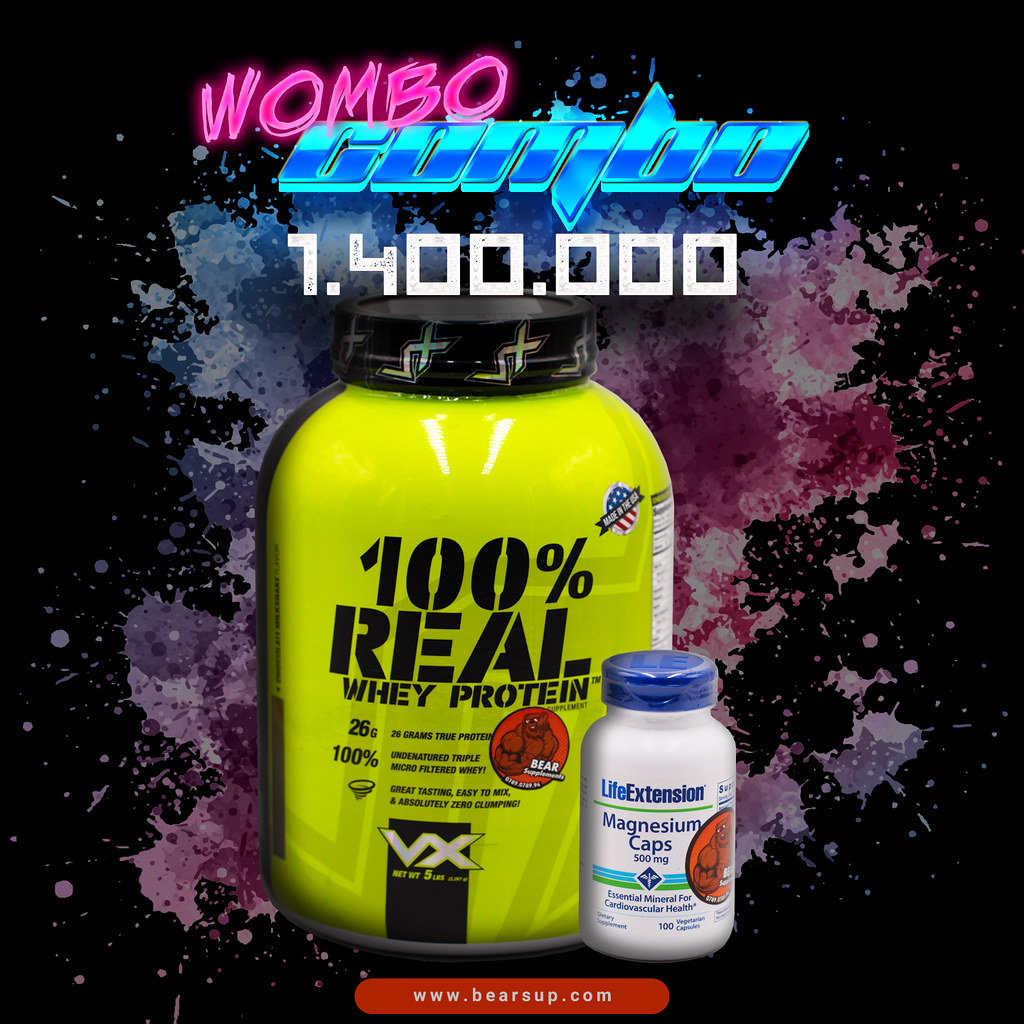The advertisement features a striking black background with dynamic splashes of pink, purple, and gray hues, creating an eye-catching backdrop. At the top, bold white text reads "Wombo Combo" accompanied by a large numeral "1.400.000" below it. Dominating the center of the image is a prominent yellow container labeled "100% Real Whey Protein." While some details on the container, including "26%", are partially obscured and not entirely readable, the product remains the focal point. Adjacent to the protein container is a bottle of "Life Extension Magnesium Caps," with a dosage of 300mg, although the fine print is difficult to discern. The advertisement concludes with the website "www.bearsup.com" displayed at the bottom.